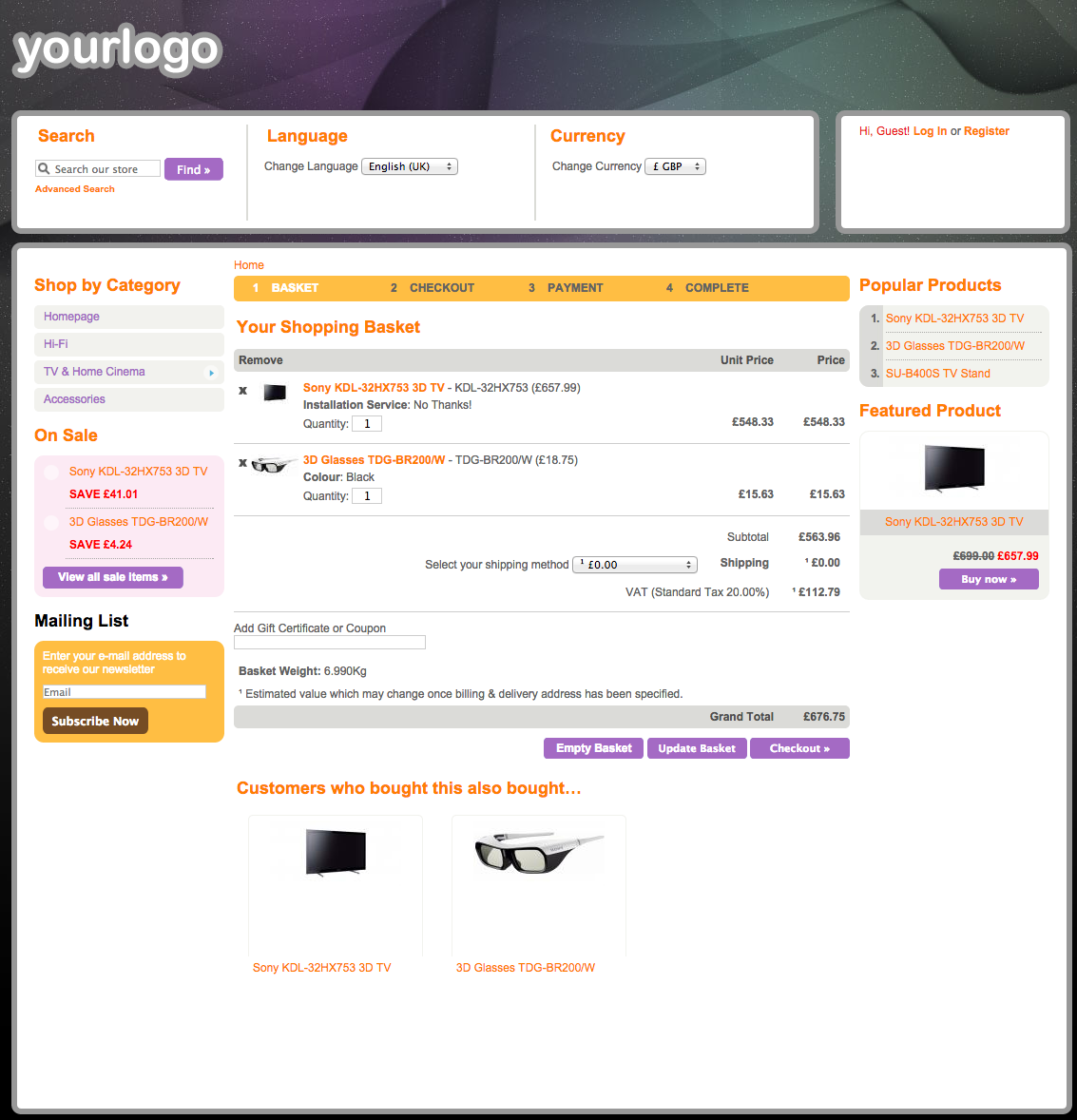The screenshot is a colorful depiction of a website. Dominating the top of the page is a black banner. On the left side of this banner, there's a white section displaying the text "Your Logo." Below this black banner lies a white section that features orange text. Moving from left to right, it says "Search" with a search bar underneath it, "Change Location" with a dropdown menu currently set to "English," and "Currency" with an option to change the currency, which is presently set to Great British Pounds (£).

On the right side of this section, the text reads "Hi Guest," followed by "Log In or Register." Below this, there's a white background showcasing a section for the user's cart or basket.

On the left-hand side of the main content section, there's a column labeled "Shop by Category," featuring menus for Homepage, Hi-Fi, TV and Home Cinema Accessories, items on Sale, and a subscription form for their mailing list.

In the center of the page, there's a rectangular, gold-colored banner that displays the stages of the shopping process: "Basket," "Checkout," "Payment," and "Complete." The current page is "Basket," showing the shopping basket contents, which include a Sony KDL and an installation service option that says "No Thank You," along with 3D glasses. The grand total for the items in the basket is £676.

On the right side of the page, there is a section for "Popular Products," accompanied by links to these items.